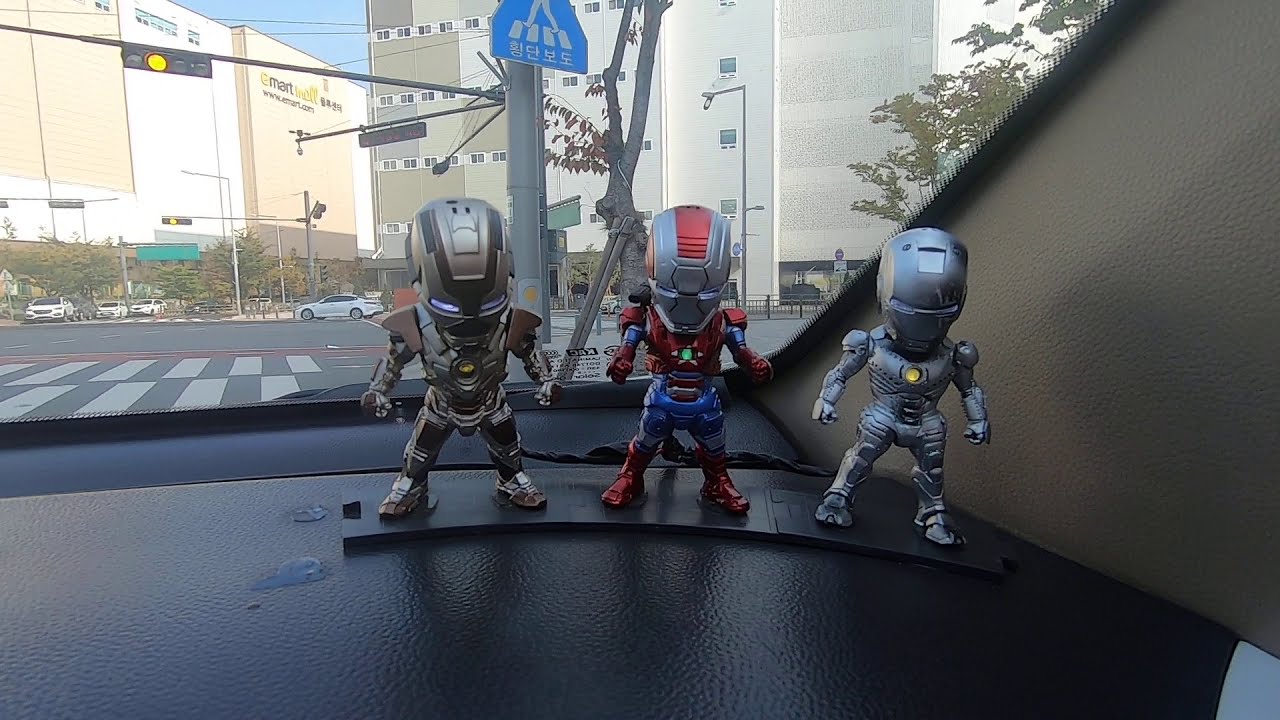In this detailed scene, three tiny robot toys are positioned on a black strip of plastic placed atop the dashboard of a car. The car’s dashboard itself is black, and the inside of the car visible on the right side has a light brown interior. Outside, through the windshield, a cityscape unfolds with several elements visible, including a crosswalk directly aligned with a stoplight showing yellow. A blue sign depicting a pedestrian crossing is mounted on the same silver pole as the stoplight. In the distance, a white car is visible on the street, flanked by multi-story buildings of various colors—light green, white, and light brown.

The robots are arranged side-by-side in center focus. The robot on the right has a mostly solid silver body with a yellow circle on its chest and is posed in an aggressive stance, its head and helmet noticeably oversized for its body. Moving to the center robot, it’s similarly postured but with more colorful detailing: it features a red helmet and shirt, green chest circle, and wears blue shorts along with blue and red boots. Its helmet has a red stripe and glowing eyes, resembling Iron Man, though distinct with different colored arms and pants, and accessorized with a small shoulder-mounted gun on its right side. The robot on the left also shares the same stance but has a darker gray palette with purple glowing eyes and distinct darker gray stripes along its hood, shoulders, arms, and legs, featuring a yellow, non-illuminated chest circle. These vivid details bring the tiny figures to life against the urban backdrop visible beyond the car’s windshield.